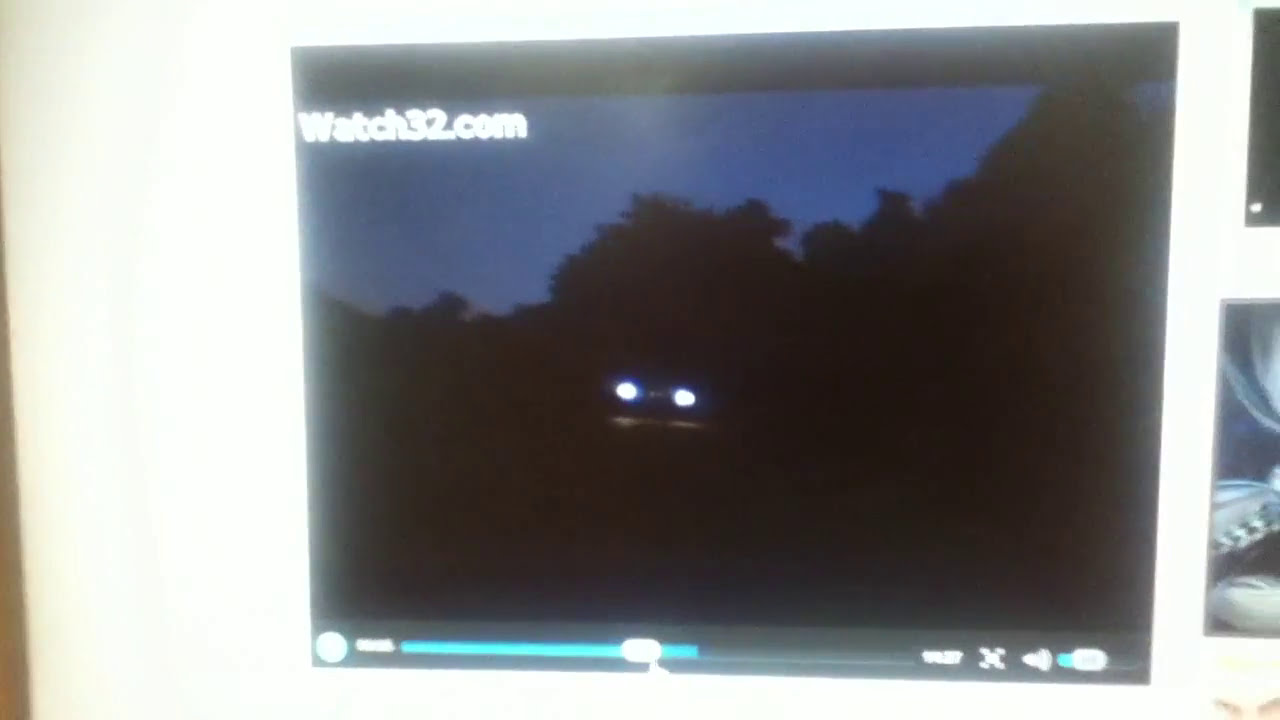This image is a blurry, color photograph in landscape orientation. It shows a freeze-frame of a video screen with a predominantly white background. At the center of the image, two headlights of an oncoming vehicle are visible, suggesting the vehicle is being driven at night or during twilight. The background features a silhouette of dark trees against a dark blue sky. In the top left corner, the text "watch32.com" is displayed in bold white letters. The bottom of the screen includes a video progress bar with a bluish line and white dots on the left, as well as a sound mute button and an 'X' icon for navigation on the right. Additionally, the right side of the image shows two cut-off screens or panels, suggesting either photographs or other video snippets. The overall style of the image is representational realism, with a strong sense of night-time ambiance despite the blurriness and some external light shining on it.